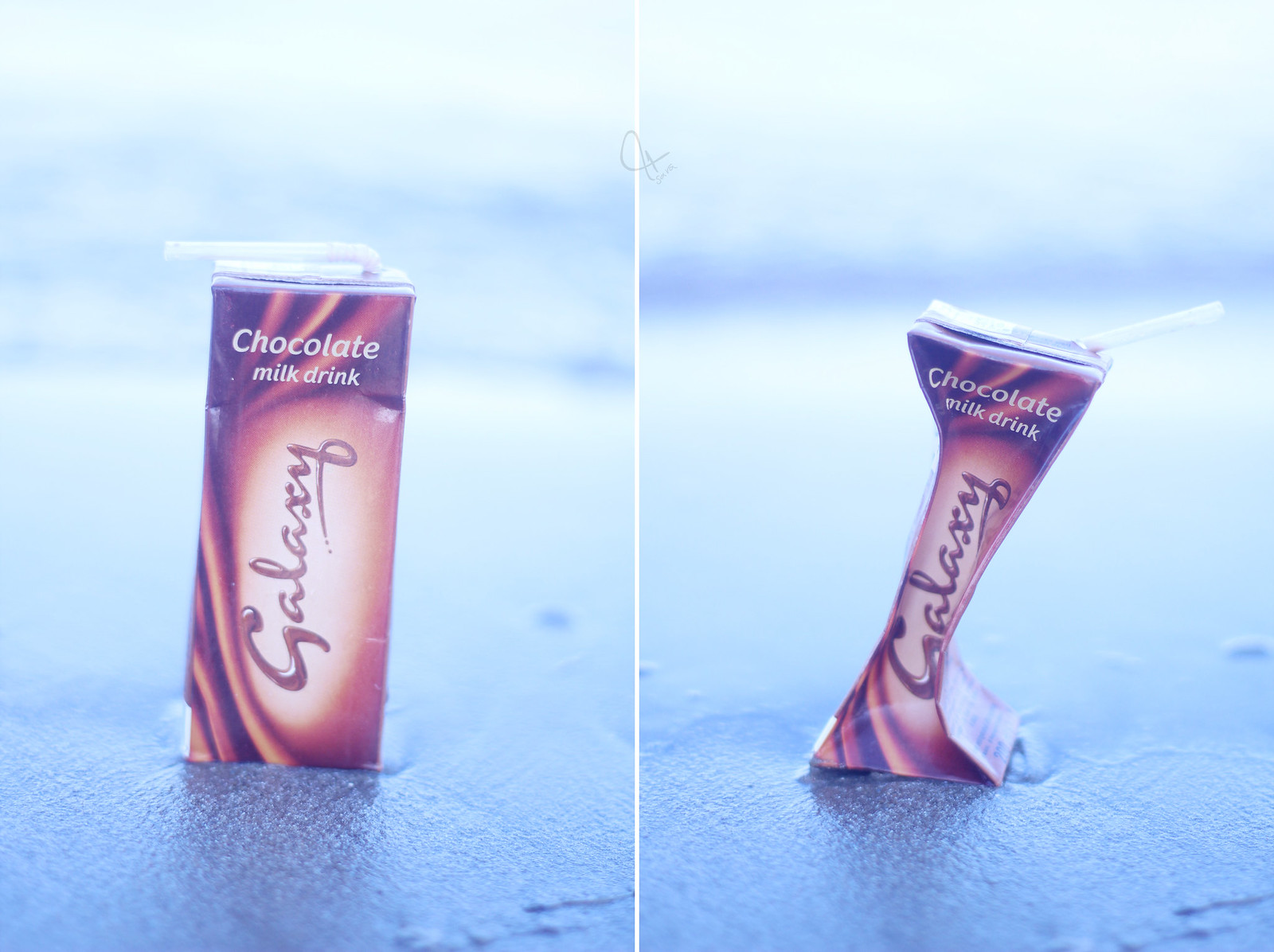In the image, there are two side-by-side pictures of a Galaxy Chocolate Milk Drink box. The left picture shows a fully filled juice box with a white straw inserted into it. The carton displays the brand "Galaxy" with beautifully designed graphics in red, purple, yellow, and brown colors, depicting a chocolate theme. The box is placed on a sandy beach surface that appears wet, possibly with ocean waves blurred in the background. The right picture captures the same juice box now empty and crumpled, tilting toward the right with the straw slightly more submerged into the carton. The sandy texture below the box and the blurred, potentially cloudy, beach background add to the scene's summery atmosphere, contrasting the states of the drink before and after consumption.